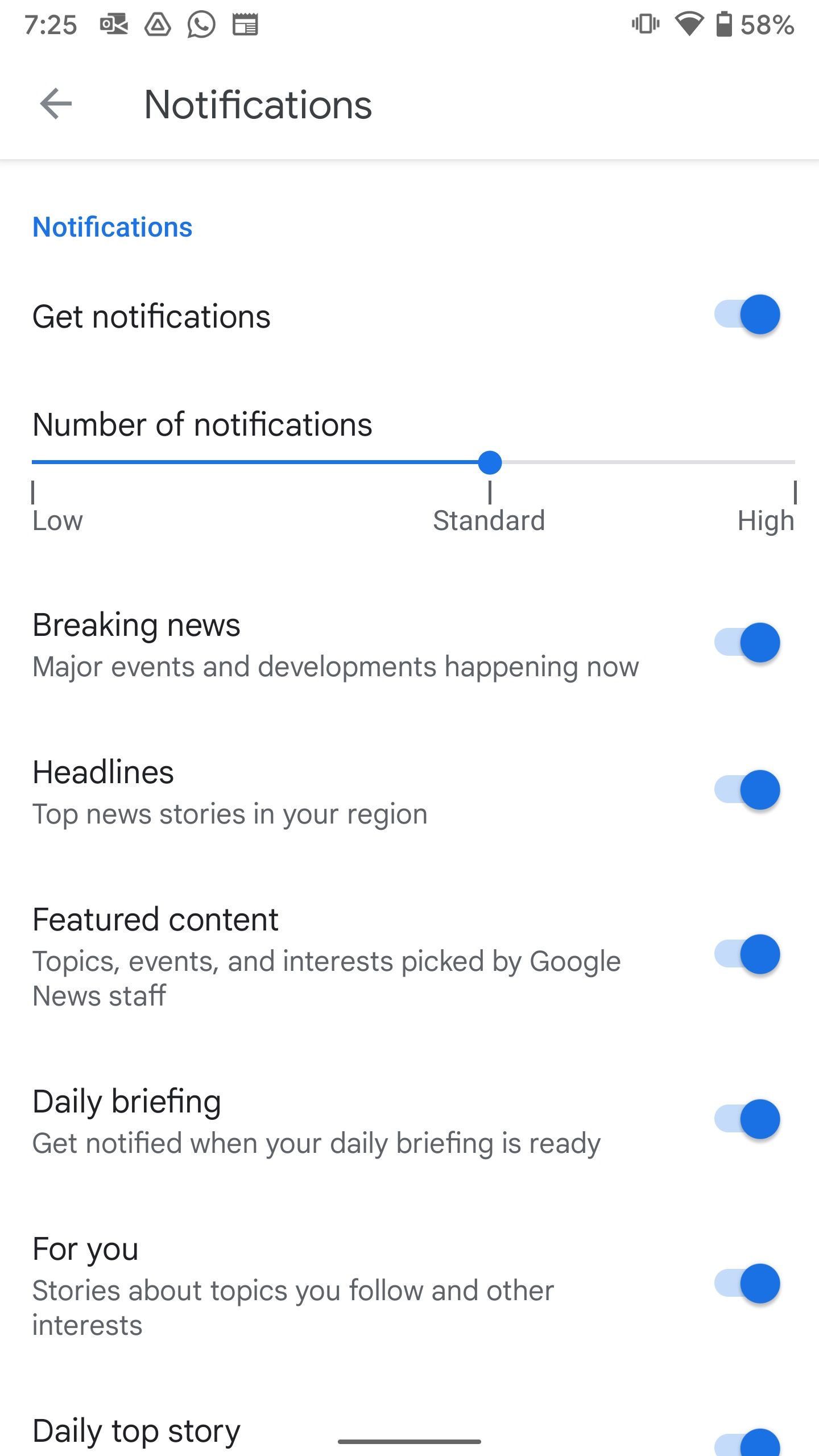The image is a screenshot of a phone screen. The battery level is displayed at 58% in the top right corner, accompanied by a battery icon. To its left, there is an icon indicating the phone signal strength, showing three or four bars out of a possible five. Further to the left, there is a vibration mode icon. On the top left side of the screen, additional icons are visible: the current time is 7:25, and there are icons for mail, Google Drive, telephone, and calendar.

Below these icons, the word "Notifications" with a left-pointing arrow appears, separated by a thin line from the section beneath it. The next section displays various notification settings in blue text, including "Get Notifications," "Number of Notifications," "Breaking News," "Headlines," "Featured Content," "Daily Briefing for You," and "Daily Top Story." Each of these settings can be toggled on or off using an oval-shaped switch, which is currently turned on, indicated by a blue circle on the right side of each oval switch. The left side of the ovals is a lighter blue.

Under the "Number of Notifications" setting, there is a bar with options labeled "Low," "Standard," and "High." The "Standard" option is currently selected.